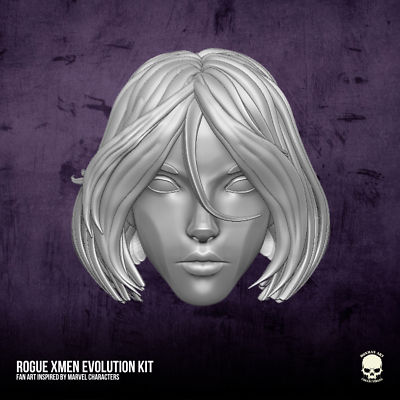The image features an intriguing and vibrant design. The background is a deep, rich purple with hues of black layered into it, creating a textured, almost scratched appearance. In the center of the image is a striking, computer-generated graphic of a silver, metallic woman's face. This face is featureless, with only angular contours hinting at the lips, nose, and eyes, which lack any pupils or whites. Her hair, also metallic in sheen, falls to her chin in a bob style, with a single strand draped down the center of her forehead over her nose. The overall look is ethereal and otherworldly. 

In the bottom left corner, white text reads "Rogue X-Men Evolution Kit," while the bottom right corner bears the phrase "fan art inspired by Marvel characters." Additionally, there is a graphic of a skull beneath the white text on the right side, adding an edgy element to the design. The image, thus, seems to be themed around the Marvel character Rogue, combining both surrealistic art and comic book elements.